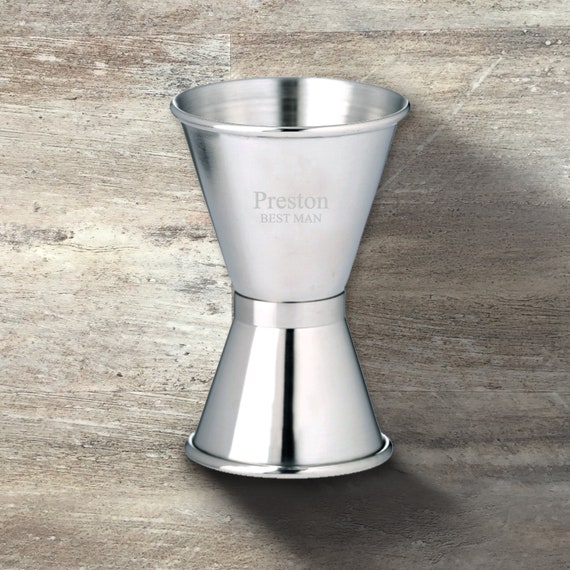The photograph features a close-up of a professionally taken shot of a shiny silver jigger, which appears to be a special gift for a wedding's best man. The jigger, almost cylindrical but with a distinctive hourglass shape, resembles two mirrored halves joined in the center by a round silver belt. The engraving on the front reads "Preston" in large letters, with "Best Man" in smaller letters beneath it. The jigger is prominently positioned against a woody, grainy background that features various shades of brown, off-white, and gray. The lighting highlights the jigger's metallic sheen, making the engraved text clearly visible. The image is clean and devoid of any other objects, emphasizing the jigger as the focal point.